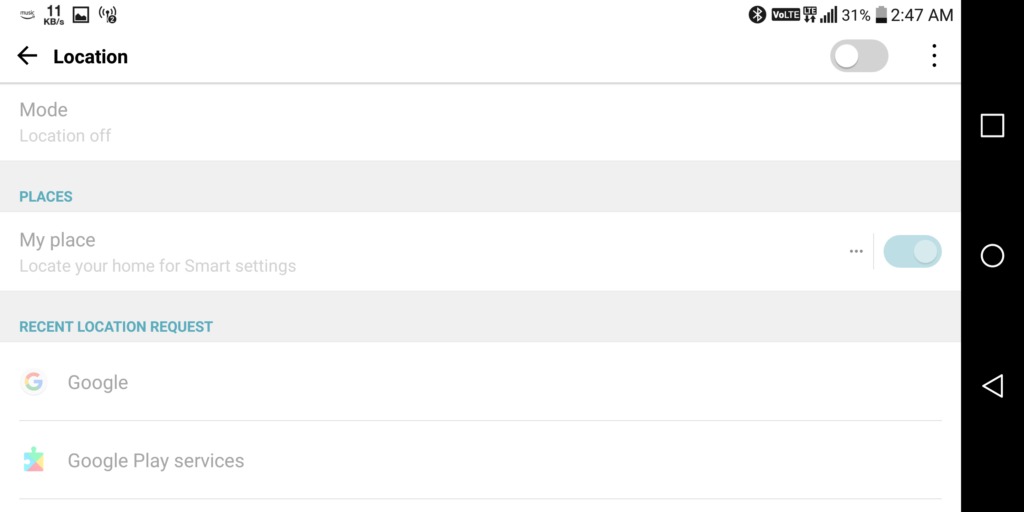This is a detailed screen capture of a smartphone interface taken at 2:47 AM. 

At the top left corner, there is a series of four gray icons on a white background, likely linked to Amazon Music—each icon being 11 KB in size, an image square, an antenna signal with a notification counter displaying "2". On the far right of this section, there is a gray Bluetooth icon, an LTE indicator, full Wi-Fi signal bars, a battery icon showing approximately 25% charge, and the time "2:47 AM".

Directly beneath these icons is a gray oval button that is toggled off. To its right are three vertically aligned black dots. On the far right side of the screen sits a black navigation bar commonly found at the bottom of smartphones, featuring a triangle, a white circle, and a white square.

In the top left, under the icons, a gray back arrow is labeled "Location". Below that, a line says "Mode" in gray. Further down, on a horizontal off-white banner highlighted in blue, the word “Places” is written. This is followed by "My place" in gray text on a white background, along with the instruction "Locate the home for smart settings". 

Towards the bottom of the screen, under the section "Recent location request," there are two entries: the Google logo accompanied by the word "Google," and the Google Play logo with the text "Google Play services."

The entire depiction captures a segment of the smartphone’s settings interface detailing location and smart settings controls, along with notifications and status indicators.